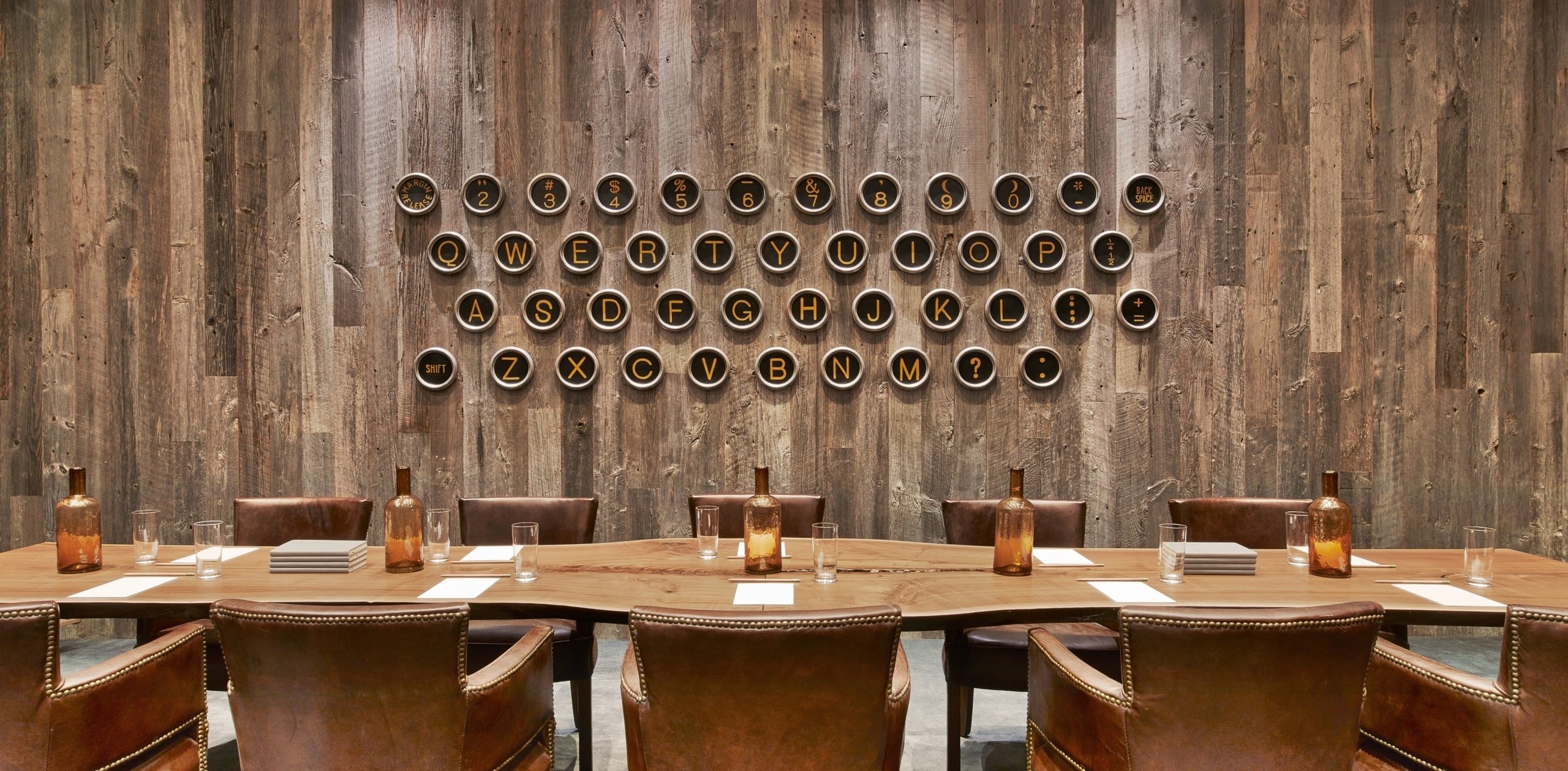This image depicts an eclectic boardroom featuring a long, brown wooden conference table that stretches from the left to the right side of the frame. The table is adorned with several items, including glass bottles—likely containing water—tan in color, and empty drinking glasses positioned at each place setting alongside white sheets of paper or notepads. Surrounding the table are large, comfortable leather armchairs. The back wall of the room is constructed from heavily-grained, unfinished-looking wooden planks that resemble hardwood flooring placed vertically. The most striking feature of the room is a massive artistic display on the back wall, comprising multiple large, circular frames that mimic the layout of a QWERTY keyboard. Each circle encloses a character—letters, numbers, or punctuation marks—set against a black background with yellow characters, evoking an old-school typewriter aesthetic. The room's cohesive wood tones and unique wall art create a fascinating blend of rustic and modern design elements.